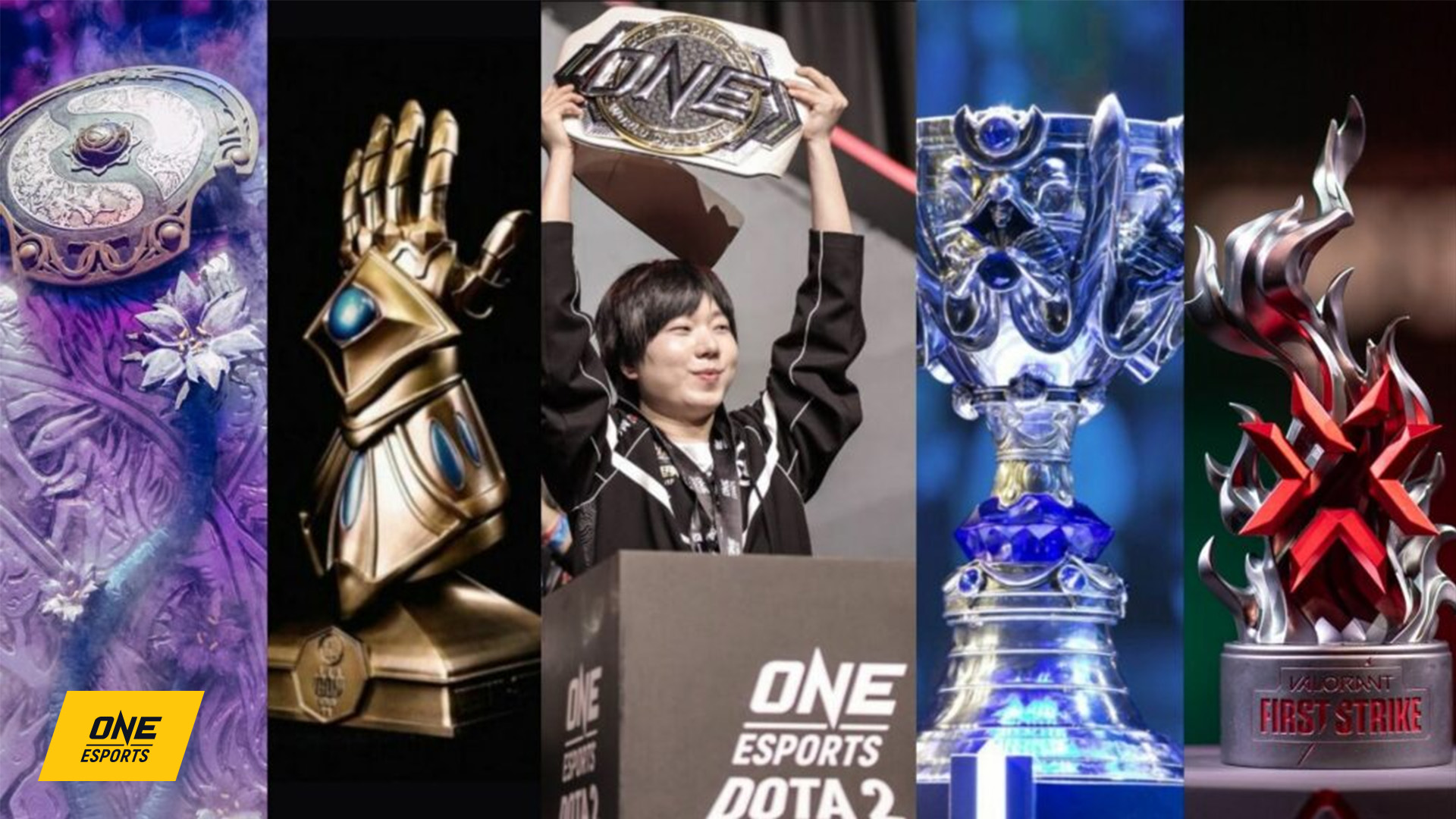The rectangular image, which is longer than it is tall, is divided into five distinct panels. 

In the leftmost panel, at the bottom, a yellow box contains the text "ONE Esports" in black letters. Above this box is a piece of silver and white jewelry, adorned with a white flower and other white and lavender figures that resemble the legs of someone sitting.

The second panel features a stark black background showcasing a golden trophy in the shape of a left hand, adorned with blue details that might be diamonds. The hand appears to be protected by a shield or cover over the forearm and rests on a golden pedestal.

The central panel displays a proud, smiling Asian woman with black, medium-length hair. She is lifting a belt or award emblazoned with the word "ONE." She wears a brown robe, and the podium in front of her reads "ONE Esports" in white letters. There is additional text that partially reads "P-O-T-E-2."

In the fourth panel, an award reminiscent of the Stanley Cup is depicted. The pedestal of this award is bell-shaped, topped with something purple. Above it sits a cup featuring an ornate design in blue, white, and purple hues.

The rightmost panel prominently features a red and silver trophy with a flame-like, pointy top. The trophy rests on a gray pedestal and is marked with the words "FIRST STRIKE" in bold, red, capital letters. 

Overall, the image is vibrant, incorporating a mix of colors including white, blue, purple, brown, gray, aqua, yellow, red, and silver. It effectively highlights various prestigious trophies and awards within the context of the "ONE Esports" theme.